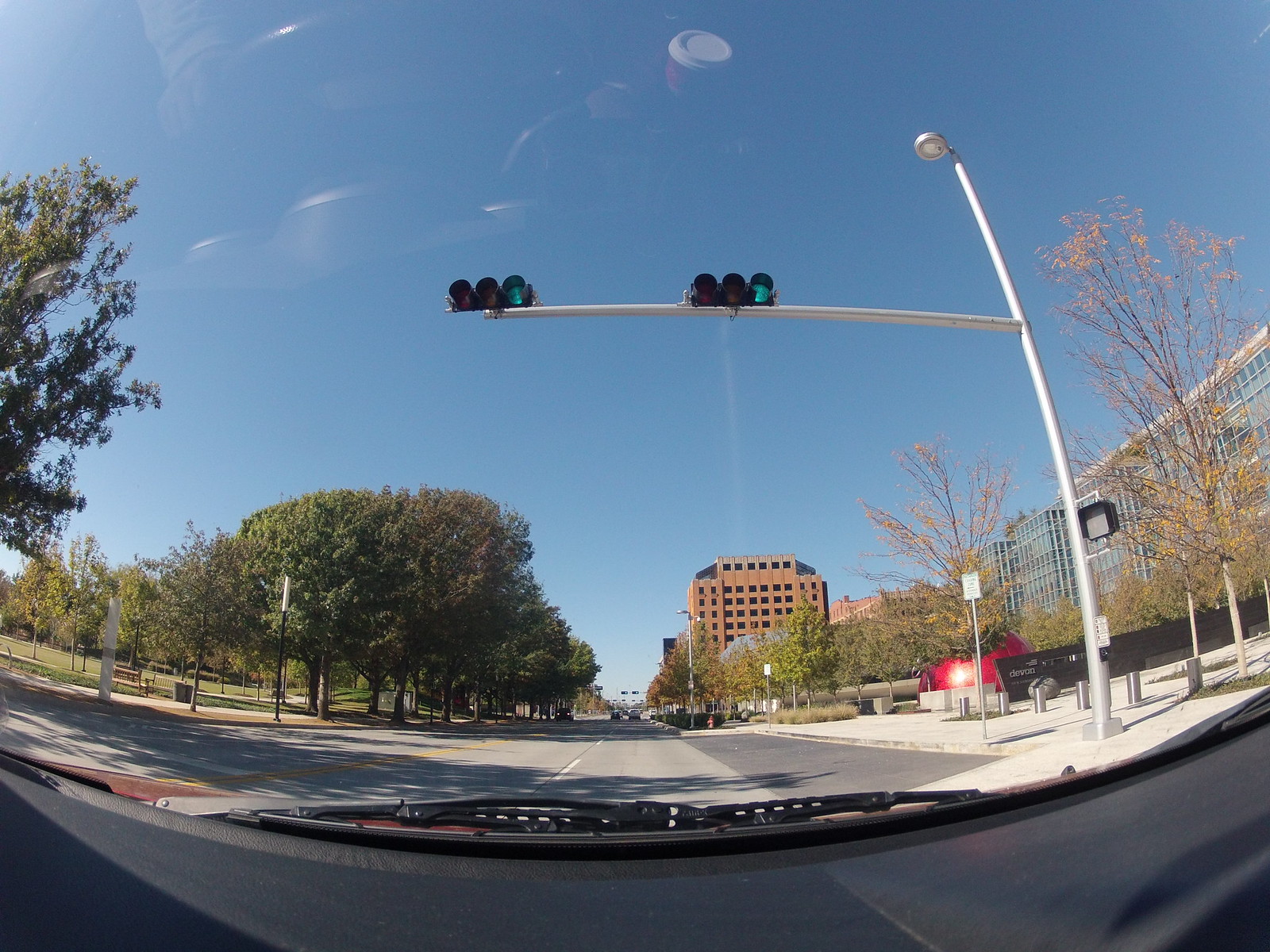This image, evidently captured from inside a car—possibly via a dash cam—offers a detailed street view through the windshield, with a slightly fish-eyed perspective. Prominent reflections of the dashboard and windshield wipers suggest a clear, bright day under a vivid, cloudless blue sky. The vehicle appears stationary at a traffic light that has just turned green, given the clarity of the scene. Dominating the view are white center lines on an asphalt road that stretches straight ahead toward a cluster of buildings in the distance, likely part of a cityscape. On the left, a lush array of green trees suggests the presence of a park or natural area, while the right side showcases a sidewalk leading to a sizable white and silver building. Further along, another large brown building is visible, adding to the urban ambiance of the distant background.